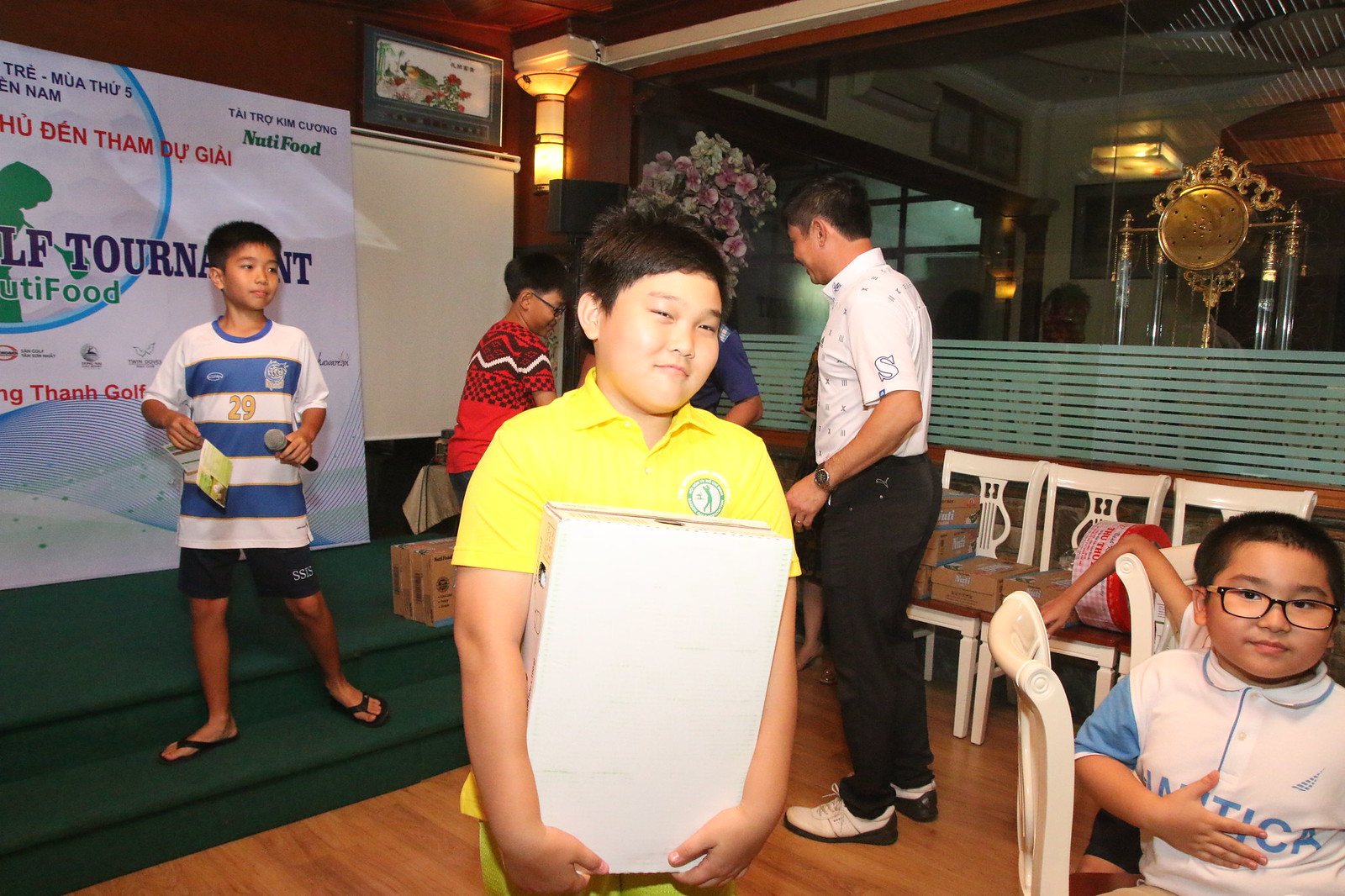This photograph captures a lively scene featuring a group of four young Asian boys, likely between the ages of 10 to 12. They appear to be in an elementary school setting in Vietnam, given the visible Asian relics and a partially legible sign indicating a "golf tournament." The boy closest to the viewer is dressed in a short-sleeved yellow collared shirt adorned with a blue logo on the right chest. Another boy stands out in a white and blue horizontally striped jersey. In the bottom right-hand corner, a boy sits on a white chair, sporting dark-framed glasses and a white collared shirt. A man, possibly in his 30s or 40s, stands in the background, though his face is not visible. The scene is set on a wooden floor with a green stage and carpet, surrounded by white chairs and cardboard boxes, with a gold metallic object hanging in the background, suggesting this could be a restaurant or an event venue.